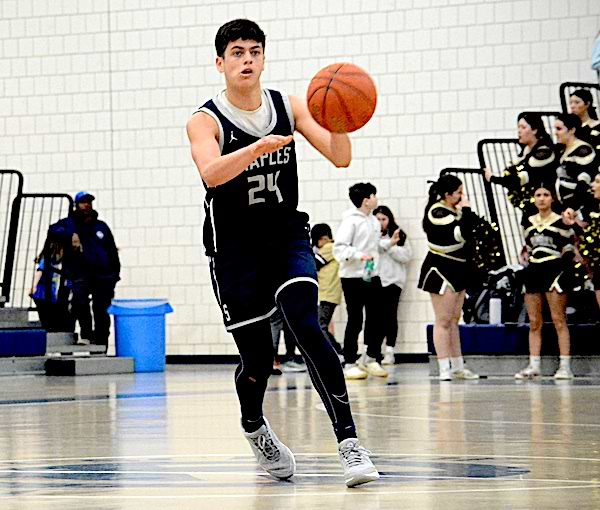The image captures a high school basketball player with short black hair, wearing a black and white jersey with the number 24 and black leggings, dribbling an orange basketball with black stripes on a tan-colored gym floor that features navy markings and white lines. The player is facing the camera, showcasing white tennis shoes. Behind him, a man, possibly the coach, stands in a coat and ball cap next to railings. To the right, a group of cheerleaders dressed in black and gold skirts cheer energetically. The gymnasium's background displays a large brick wall made of white tiles, and to the left, a blue barrel trash can is visible. The setting suggests an engaging high school basketball game, with various spectators and participants positioned as expected – standing, sitting, and actively engaged in the game.